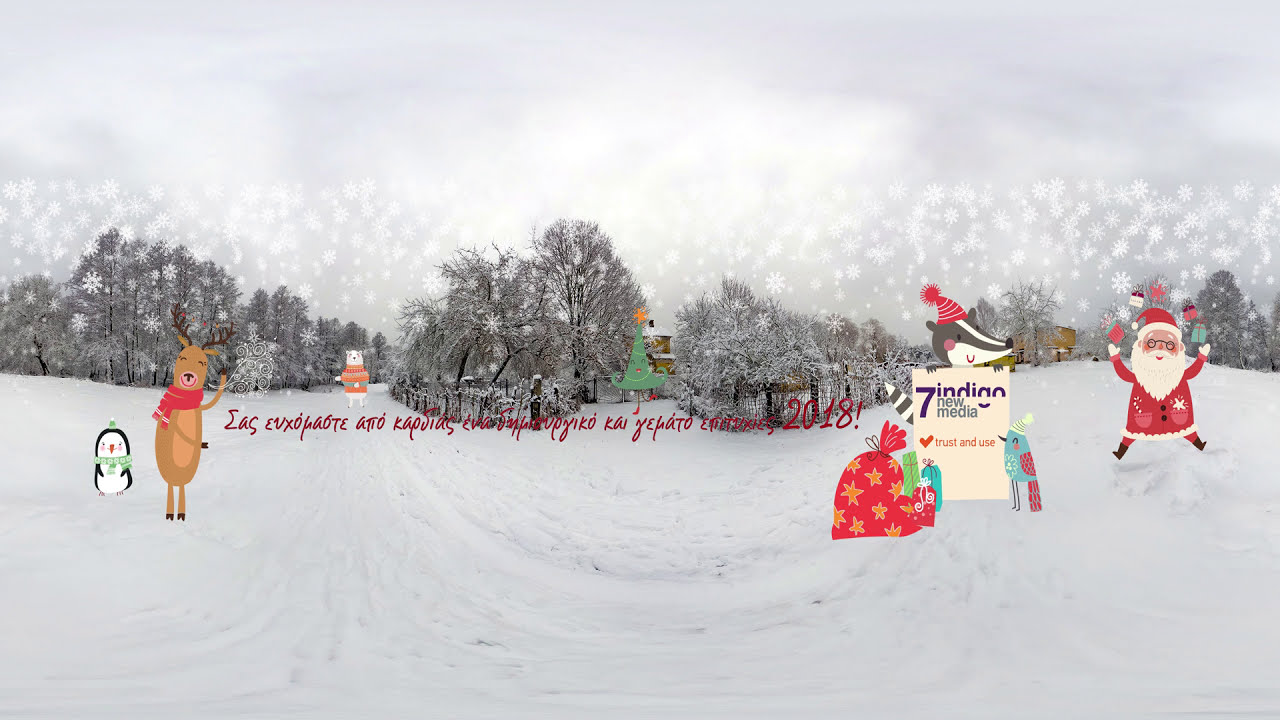The image depicts a festive Christmas scene combining a wintry forest photograph with overlaid cartoon graphics. The snowy background features an overcast sky, barren trees with snow-laden branches, and a partially obscured golden building. Snow blankets the ground, which shows trails from tire tracks or a sled.

Overlaying the photograph, there are several animated characters and festive elements. Starting from the left, a cute black and white penguin stands next to a smiling, waving reindeer, adorned with dark brown antlers and a red scarf. Towards the background, a polar bear in a sweater can be seen. Centered in the image is a decorated Christmas tree with a star atop it and several colorful presents. To the right, a skunk wearing a Christmas hat holds up a card that reads "7 Indigo New Media Trusted Use," with a bird gazing at the sign and smiling at it. Farther right, Santa Claus, jubilant and dressed in his traditional red suit with a white beard and glasses, appears to be juggling gifts.

Snowflakes fall throughout the scene, enhancing the festive atmosphere. At the top of the overlay, red text, difficult to decipher due to being in Greek, shares a message that includes "2018!" with an exclamation mark, indicating the year. The overall vignette beautifully merges the charm of natural wintry beauty with whimsical holiday cheer.